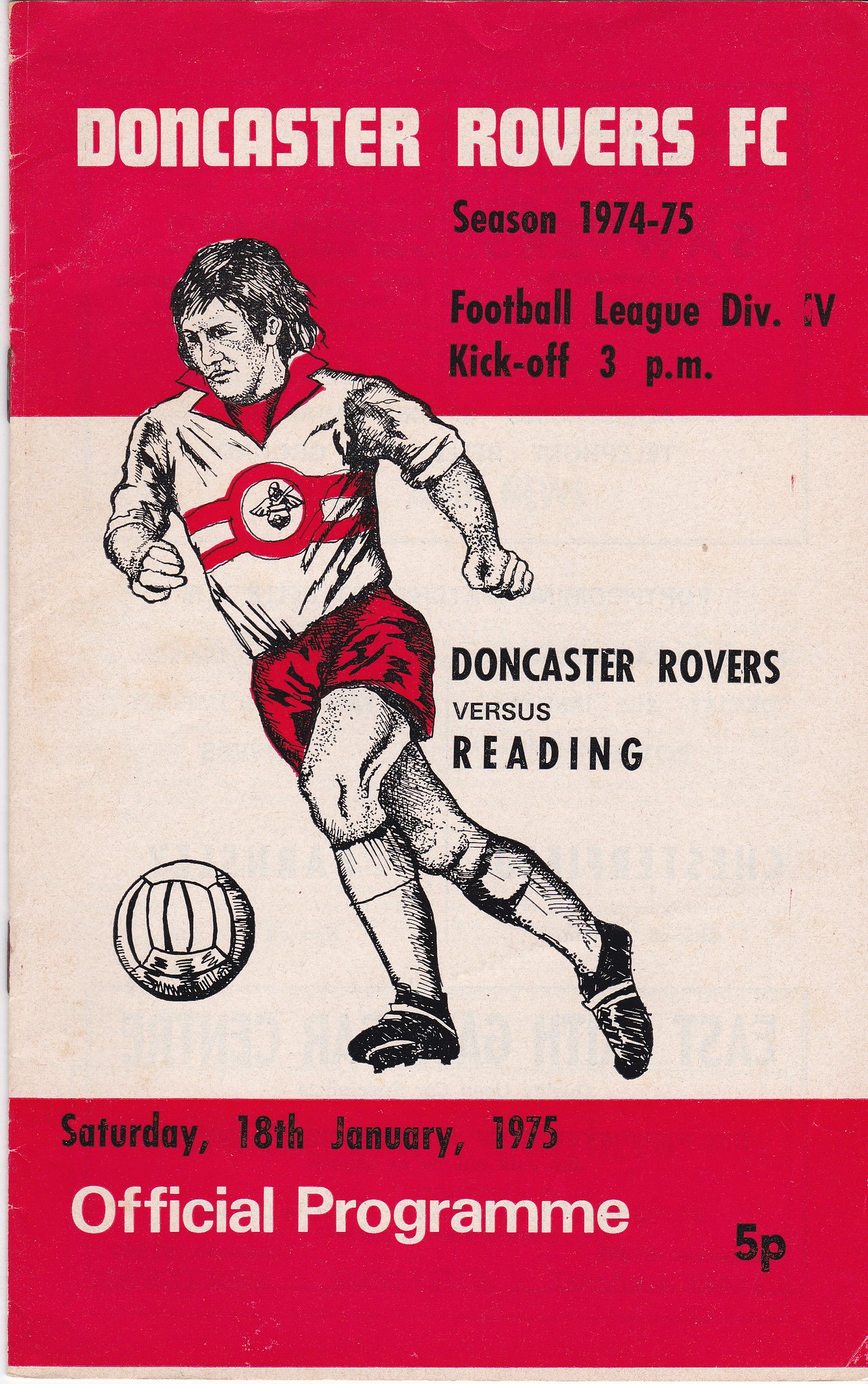This image depicts a cover from an old official program of the Doncaster Rovers Football Club, a European soccer team. The top of the red and white program prominently displays "Doncaster Rovers FC" in white letters. Directly beneath, black text reads "Season 1974-75, Football League Division 4, Kickoff 3pm." The center shows a detailed black and white sketch of a soccer player in motion, wearing a uniform with a white jersey featuring red stripes and a red circle containing the team logo, along with red shorts and cleats. To his right, the text "Doncaster Rovers vs. Reading" is printed in black. Below, the date "Saturday 18th January 1975" appears in black lettering. In the bottom right corner, "Official Programme" is written in white, accompanied by the price "5p" in black.